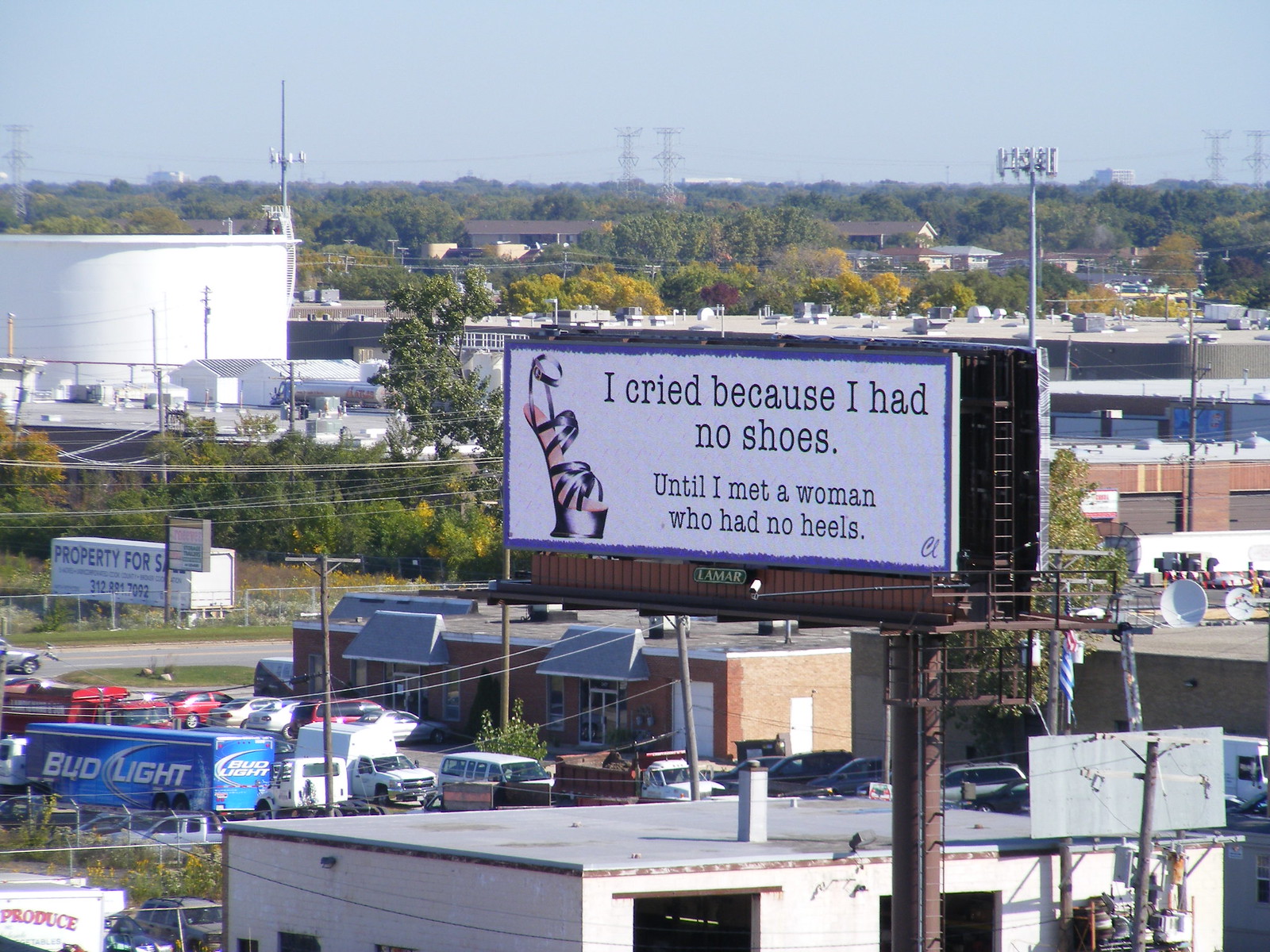This aerial photograph captures a bustling urban landscape, characterized by a mix of commercial and industrial elements. Prominently featured is a Lamar billboard, situated tall and central in the composition, likely the focal point of the image. The billboard, supported by a sturdy brown pole with an attached ladder, conveys a poignant message in bold white text against a blue border: "I cried because I had no shoes," followed by a smaller-font continuation, "until I met a woman who had no heels," accompanied by an image of a high-heeled sandal.

In the background, a Bud Light semi-truck, colored in blue and white, is visible among an array of buildings, highlighting the commercial activity in the area. The distant cell phone towers and towering silver and gray electrical lines add to the urbanity of the scene. The photograph is rectangular and provides an expansive view, offering a detailed glimpse into the elements that makeup this lively cityscape.